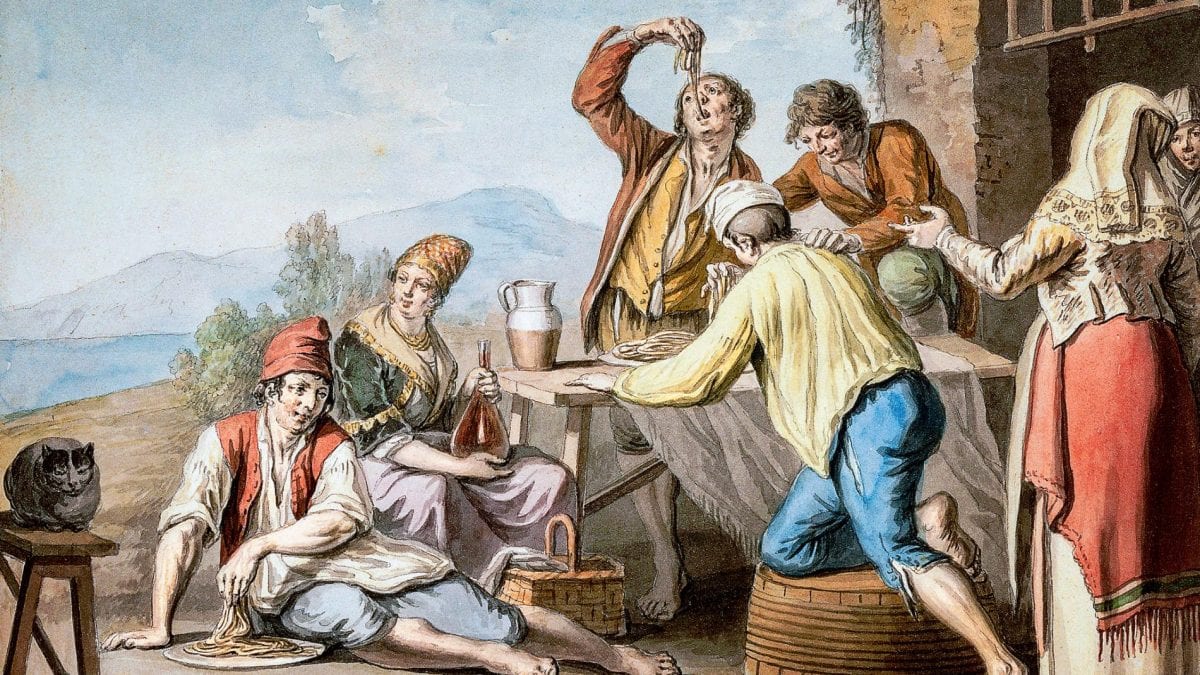A detailed illustration, likely from pre-Renaissance Europe, showcases a lively scene with seven individuals gathering around a wooden table, devouring pasta with their hands. Set against a backdrop featuring sketched mountains and a serene sky adorned with white clouds, the vivid scene bustles with life. On the left, a black cat perches on a brown wooden bench. Closest to the viewer, a barefoot man with a red cap, vest, and knee-length blue pants sits on the ground, his hand diving into a bowl of pasta. Adjacent to him stands a woman, adorned in a gold hat and a beige-trimmed green top with a long skirt, holding a jug and gazing off over the man's head.

At the table's center, another man, dressed in a gold shirt and rust-colored jacket, stands and holds a string of pasta above his head, stuffing it into his mouth, while a woman beside him in similar gold attire also reaches over to grab pasta. To the right, a barefoot man with a yellow shirt and blue pants reaches over the table, his back turned to the viewer. In the foreground, a woman in a long red skirt and beige top stands with her back to the viewer, one hand outstretched in a gesture. The scene, accented by a distant building and possibly a lake or seaside, is rendered in a colored pencil style. Despite its historical semblance, it is notable for its anachronistic details, hinting it may be an AI-generated image.